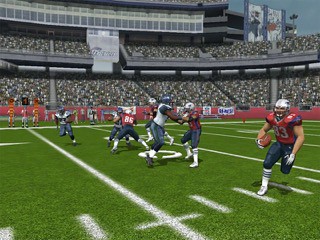This image is a screenshot from a video game depicting an intense moment on a football field. Dominating the scene is an intricately rendered pitch with several players positioned strategically across it, showcasing the game's realistic and detailed graphics. On the right side of the image, a player in a muted red jersey and slate gray pants rushes toward the viewer, adding a dynamic sense of motion. Centrally located, two of his teammates can be seen preparing for action.  Opposing them are two players in white jerseys, adding contrast to the scene. In the background, a densely packed stadium filled with spectators adds to the atmosphere, reinforcing the game's lifelike realism despite the clearly digital rendering of the characters.